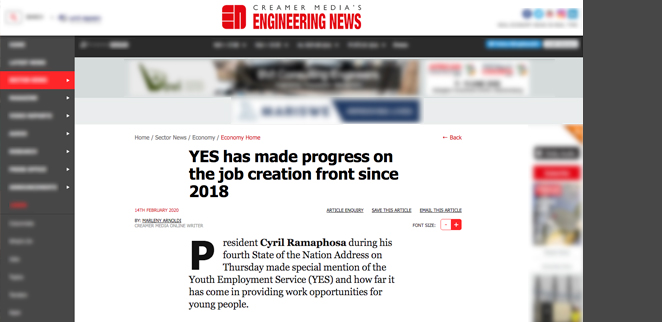Screenshot of a website with a Creamer Media’s Engineering News banner at the top center. The background features a mix of black and gray areas with blurred text on both the left and right sides, as well as across the top, making the text unreadable. There is a red-highlighted clickable element near the top left, but its content is also indiscernible due to the blur. 

The central portion of the image showcases a white section with black text that reads: "Yes has made progress on the job creation front since 2018. President Cyril Ramaphosa, during his fourth State of the Nation address on Thursday, made special mention of the Youth Employment Service, YES, and how far it has come in providing work opportunities for young people."

The background contains more blurred elements with various colors and words, creating a visual impression reminiscent of a store environment.